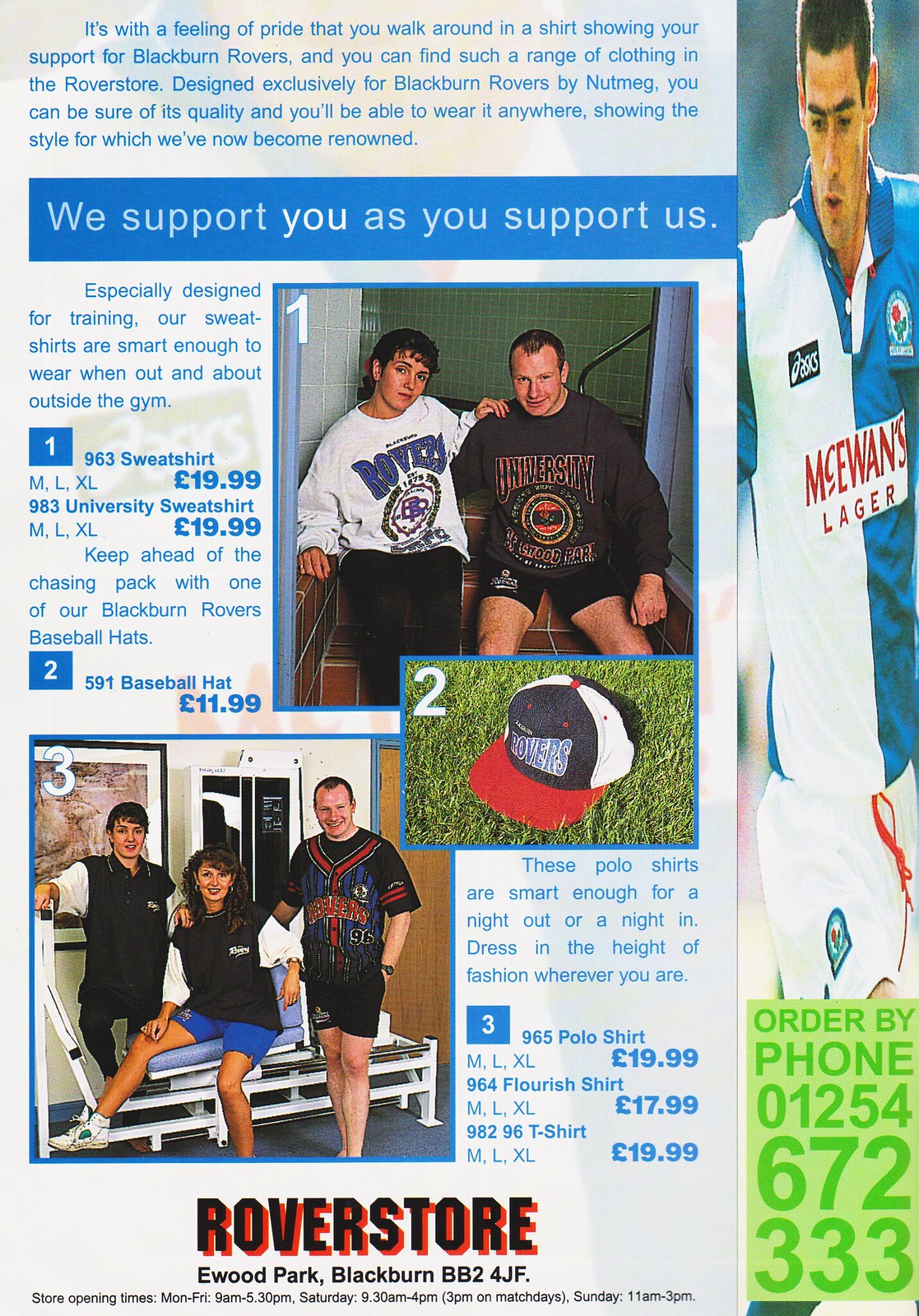This advertisement showcases the exclusive range of Blackburn Rovers merchandise available at the Rover Store. Prominently featuring a man in a sports jersey poised to kick a ball, the right edge of the ad highlights the tagline "Order by phone, 012-5467-2333." The ad emphasizes the pride and style of supporting Blackburn Rovers, with a blue banner stating, "We support you as you support us." 

The central section of the advertisement details various apparel options, including sweatshirts, polo shirts, and baseball hats, indicating the sizes (medium, large, extra-large) and prices (sweatshirts and t-shirts for L19.99, hats for L11.99, polo shirts for L19.99, flourish shirts for L17.99). 

Visual elements include a picture labeled number one of someone in a Rovers t-shirt, a picture labeled number two featuring a Rovers baseball hat on green grass, and a picture labeled number three that shows two women and one man modeling Rovers polo shirts. Another image displays two men wearing sweatshirts, one in black pants and the other in black shorts, representing the smart yet functional design of the apparel suitable for both training and casual wear.

At the bottom of the ad, the Rover Store location is specified as Ewood Park, Blackburn, BB2, 4JF, with store hours listed for convenience. Overall, the ad promises quality and fashionable clothing for Rovers fans, designed by Nutmeg and showing the club's renowned style.